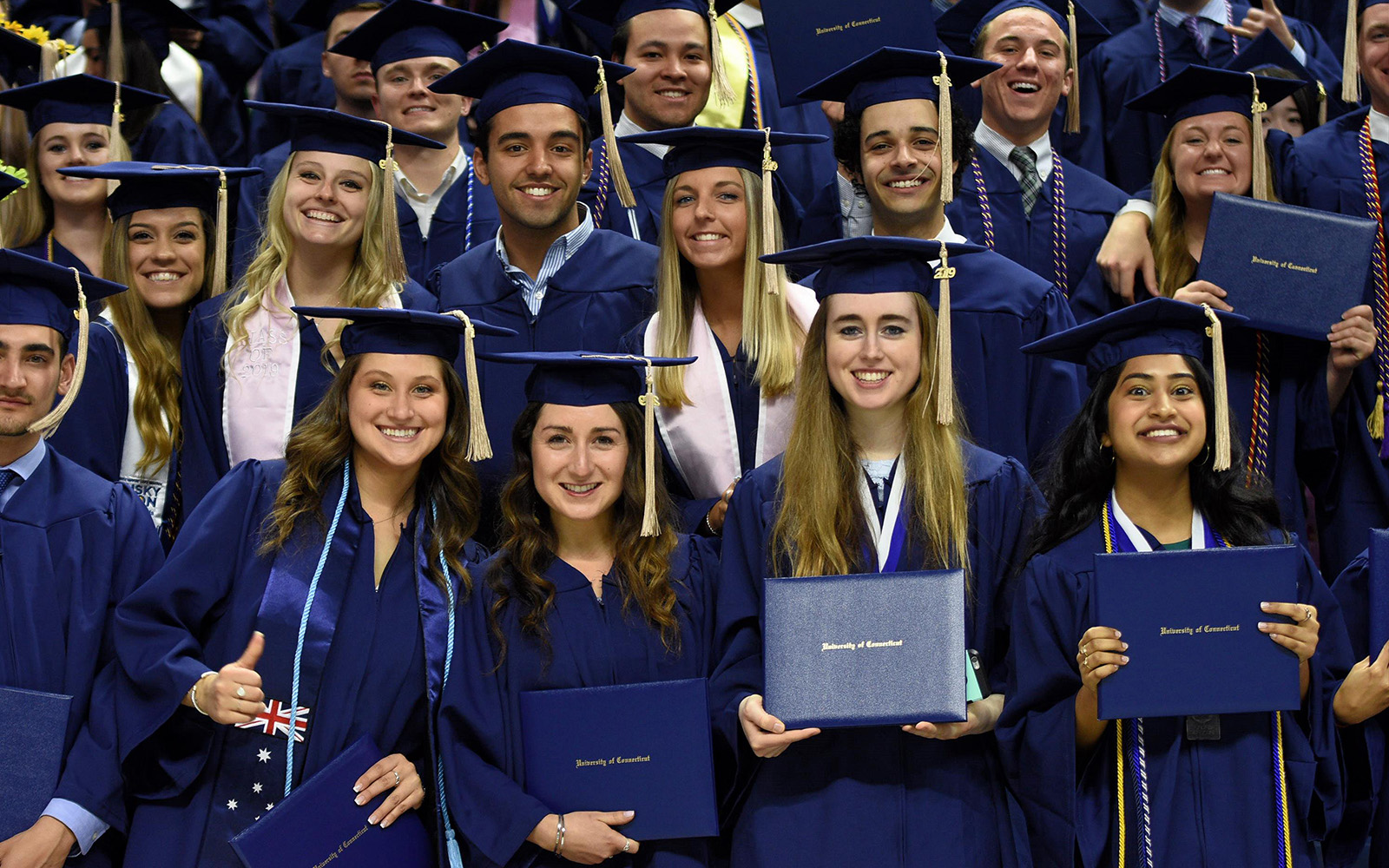The image depicts a vibrant group of approximately 20 high school or college graduates from the University of Connecticut, all smiling brightly at the camera. The students, a diverse mix of males and females, are arranged in three visible rows and are dressed uniformly in dark blue caps and gowns. Each cap features a square board topped with a gold tassel, and some students are adorned with medals. Several graduates in the front row proudly hold their dark blue diplomas with gold text. Notably, a woman on the left stands out with a blue scarf bearing the British flag, although earlier descriptions mentioned an Australian flag. Some students in the middle are wearing white scarves, while others sport sashes or braided cords of gold. This group exudes joy and pride, captured in a moment of celebration.